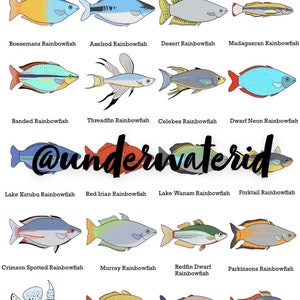The poster features an array of animated cartoon fish, organized into 5 rows with 4 fish in each row, totaling 20 fish. Each fish is brightly colored and diverse, showcasing different types of rainbow fish with unique patterns and hues ranging from light greens and blues to vibrant reds and oranges. Every fish is labeled with its scientific name. Prominently displayed in the middle of the poster, overlapping the third row of fish, is the cursive black text reading, "At Underwater ID." All the fish are uniformly facing to the right. The top left fish is a striking half-orange, half-light blue Bozeman's Rainbow Fish. Each subsequent fish continues to add to the colorful display, including notable ones like a gray Desert Rainbow Fish and a turquoise fish with red fins. The variety and elegant designs of these rainbow fish with their distinctive fins make for an educational and visually appealing spectacle.